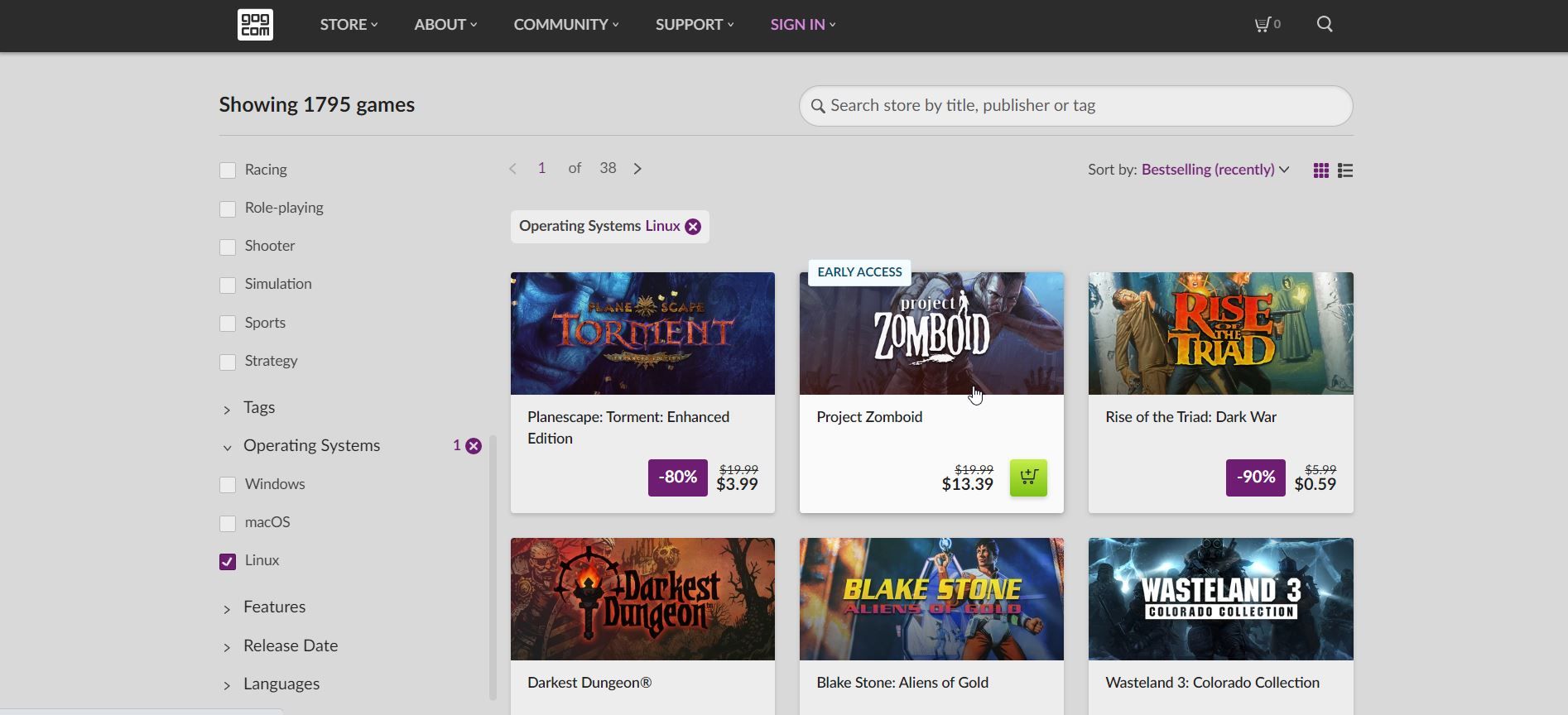The screenshot features a gray background with various interface elements visible. The top section includes options like "Store" and "Community," with the "Support" and "Sign In" buttons highlighted in purple. To the right, there is a white shopping cart icon and a magnifying glass icon, also in white. The screenshot indicates a collection of 1,795 games and includes a prominent search bar with another magnifying glass icon. The search bar is labeled "Search Store" and allows filtering by title, publisher, or tag. 

Below the search bar, there is an option to sort the games by "Best-Selling (Recently)." The display shows a grid consisting of three rows of items. Each row includes icons – purple dots, green squares, and gray rectangles. Pagination controls are present, with "1 of 38" displayed between left and right arrows, enabling navigation through the grid.

On the left side of the interface, there is a filter list that includes categories such as "Racing," "Role-Playing," "Shooter," and "Simulation." To the right of these categories, the operating system is specified as "Linux," displayed in purple text with a corresponding purple circle and a white "X." Six games are highlighted for the Linux platform, with one game at the top featuring a white rectangle with the label "Early Access" in green.